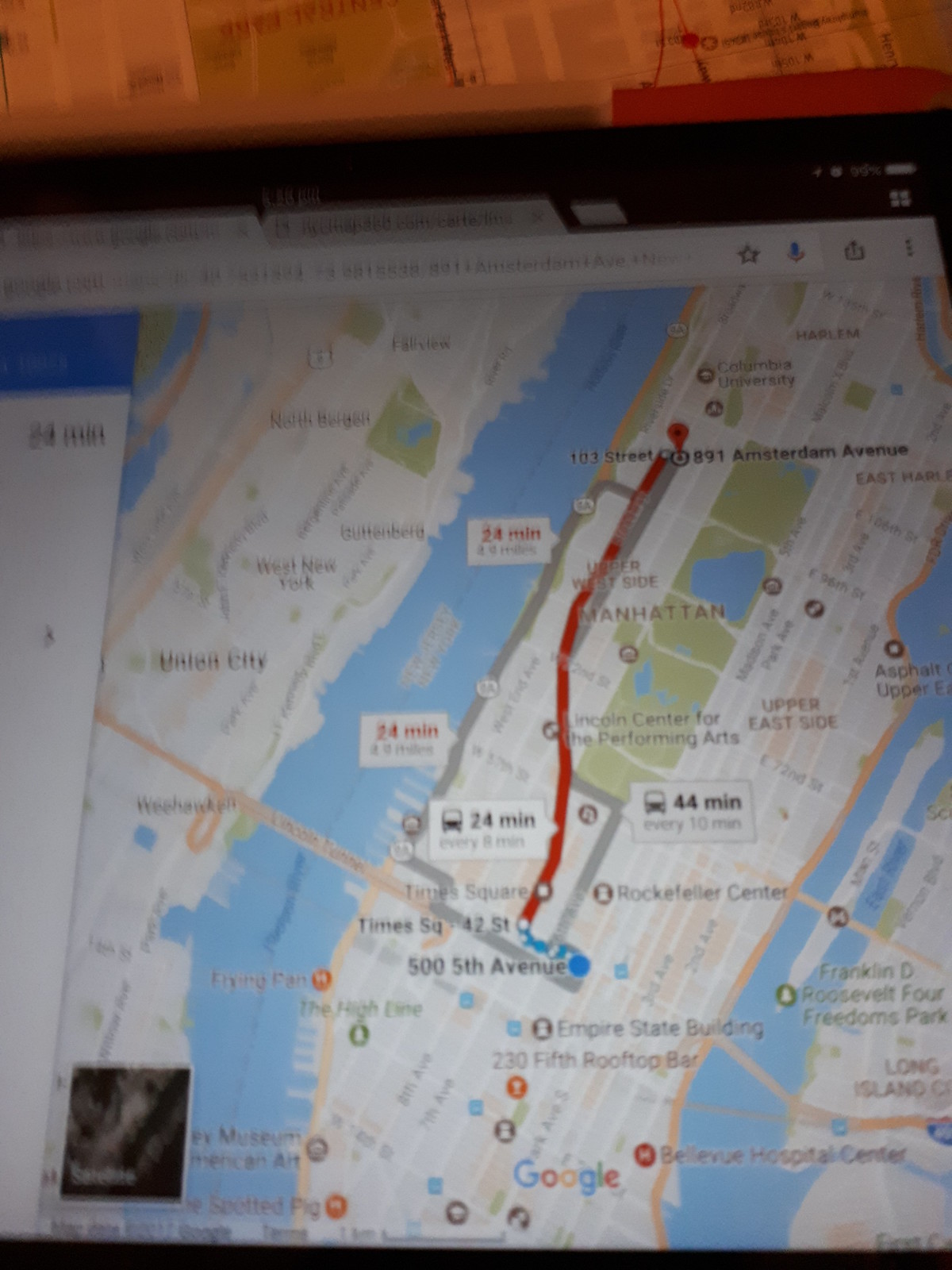This photograph captures a Google Maps image displayed on a laptop screen, taken using a phone camera. In the background, a physical map is partially visible, adding context to the digital navigation scene. The laptop's battery icon in the top right corner shows a near-full charge at 99%. The browser window has two open tabs, indicating multitasking.

The map on the screen details a route from 505th Avenue to 103rd Street, specifically 891 Amsterdam Avenue in New York City. A straight red line, signifying congestion, traces the path down Manhattan. To the left of the map, Union City is partially visible, hinting at the broader geographic context. Manhattan, bordered by two rivers, is distinctly waterlocked, with numerous markers indicating various important locations. A large park runs down the middle of the island, likely referring to Central Park.

On the left side of the screen, the navigation panel is cut off but partly readable, revealing that the journey to the destination will take approximately 24 minutes. The detailed map reflects the urban density and intricate transportation network of New York City.